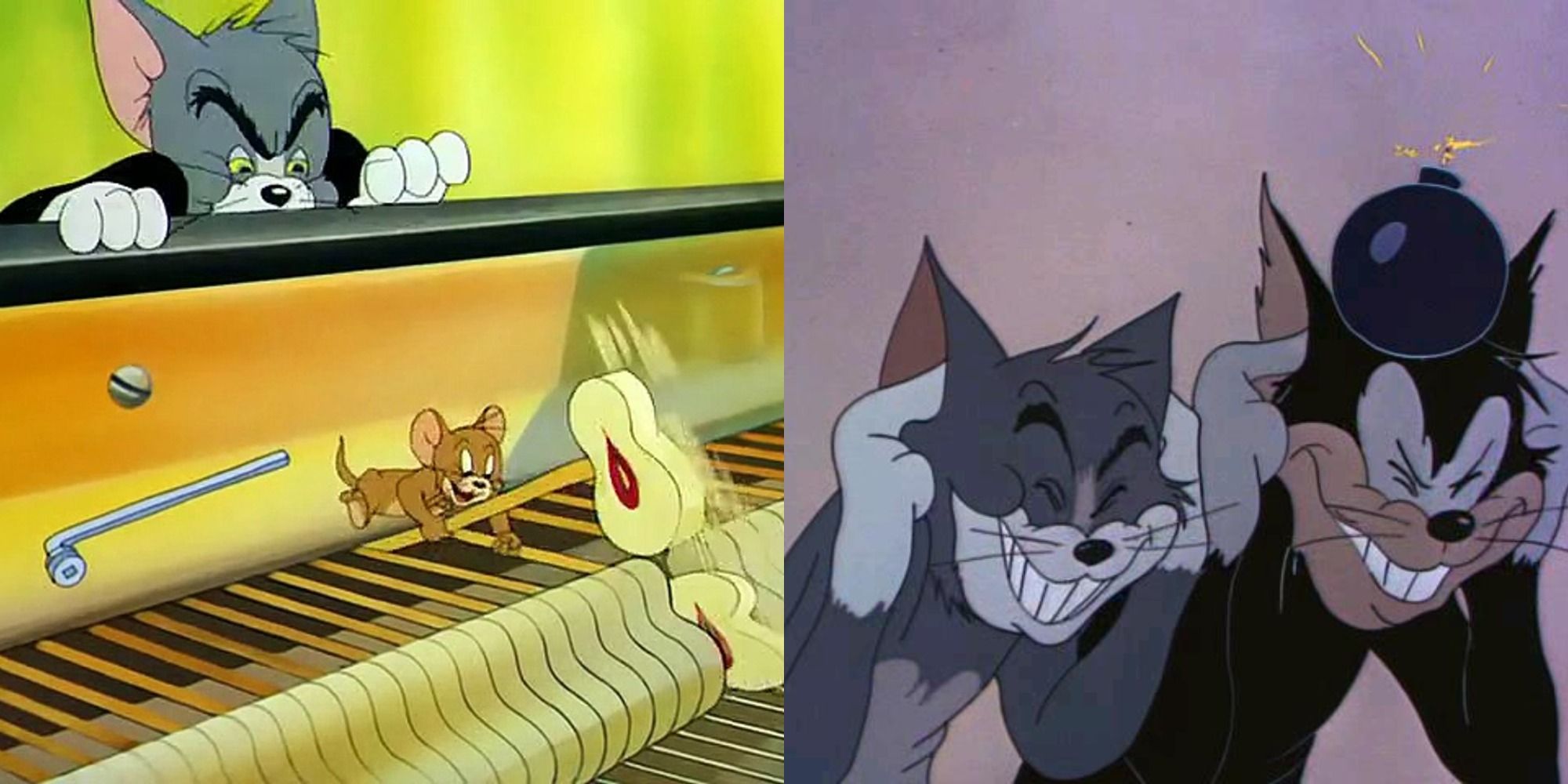This illustration from the Tom and Jerry cartoon is divided into two scenes. The left side features a mischievous Jerry the mouse inside a grand piano with a tan interior and white strikers. He's smiling as he tugs at the piano hammers, causing playful chaos. The gray tomcat, Tom, peers over the top of the piano with an aggravated and sinister expression, seemingly plotting his next move. The right side depicts Tom and an unidentified black cat, both of whom have their fingers in their ears and eyes squeezed shut. They wear smug grins as they unknowingly await the explosion of a hissing bomb that rests precariously on the black cat’s head. The background for both scenes is a vivid pink, contrasting with the darker tones of the characters and the black piano that occupies part of the left scene.